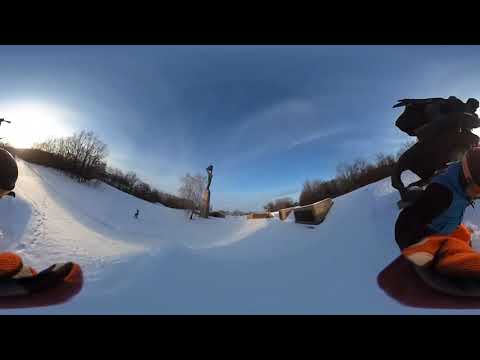This outdoor photograph captures a striking snowy landscape under a brilliant blue sky with wispy white clouds. The sun shines pale from the left side, casting gentle light across a wide, snow-covered valley that resembles a snowboarding half-pipe. The U-shaped slopes rise up on either side, flanked by bare, leafless trees indicative of winter. In the foreground, the image prominently features individuals engaged in snowboarding, with one person on the right dressed in a vivid orange and blue ski suit and a crash helmet. Their board cuts through the snow as they navigate this expansive, playful terrain. The valley's white expanse is punctuated by more colorful winter gear-clad snowboarders in the distance. A striking feature in the background is a tall monument of a human figure holding up an object, standing proudly atop an elevated pedestal, adding a unique landmark to the serene winter scene.